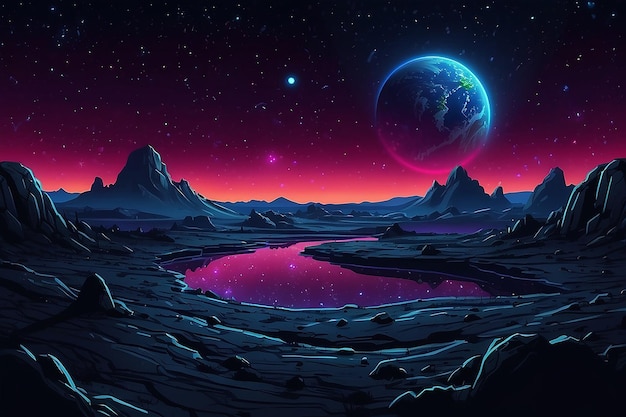The image is a detailed, computer-generated space scene illustration depicting a barren and dark rocky landscape, almost like a black desert terrain. The mountains and rock outcroppings are silhouetted in black and dark grayish-blue hues, suggesting a nighttime setting. In the midst of this dark landscape lies a reflective body of water, possibly a lake or puddle, creating a striking "C" shape that mirrors the vivid colors of the sky above.

The sky itself transitions from a star-studded black canopy at the top to an otherworldly, almost alien sunset near the horizon, blending vibrant shades of purple, hot pink, and bright orange. The top right-hand side of the sky prominently features an Earth-like planet, glowing ethereally against the cosmic backdrop, resembling the size of the moon as seen from Earth. Accompanied by what could be the Earth's own moon and a striking blue star, this celestial scene adds depth and intrigue to the illustration. Overall, the image evokes a sense of an alien world, with its stark and dramatic interplay of light and landscape.